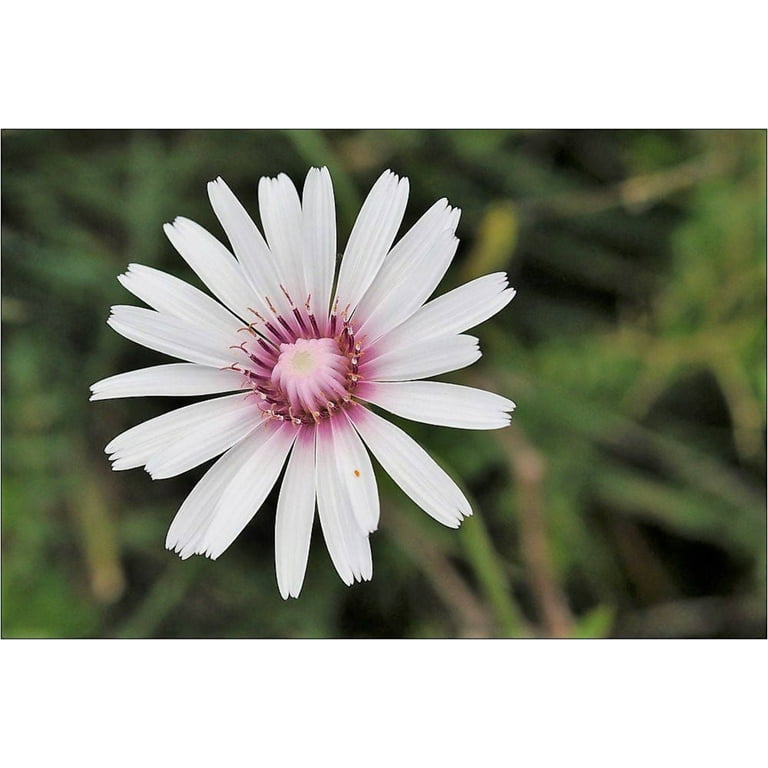The image captures a blooming white flower, resembling a daisy, in sharp focus against a blurred green backdrop of leaves or other plant life. The flower's circular shape is defined by approximately 20 thin, long petals, each with jagged edges, creating subtle gaps in between. The center of the flower stands out with a striking pink hue, transitioning into a yellow bud surrounded by delicate, pinkish-purple stamen that have golden tips. These intricate details highlight the flower's peak bloom, suggesting the photo was taken in the spring or summer season, capturing the essence of this vibrant and mesmerizing blossom amid a lush, indistinct background.